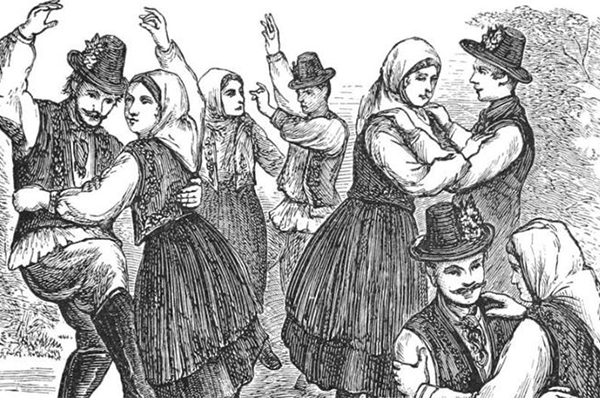This detailed black ink etching, likely from the early 1600s, portrays a lively scene of four couples engaged in traditional European dance, reminiscent of Bavarian Oktoberfest attire. The men are adorned with dark black hats and most sport mustaches, while the women uniformly wear white kerchiefs around their heads and long black dresses. Two of the couples raise their hands jubilantly in the air, while the other two dance more traditionally, with one gentleman holding his partner tightly. The background features sketched foliage, including trees and bushes, enhancing the rustic, pastoral setting of the scene.